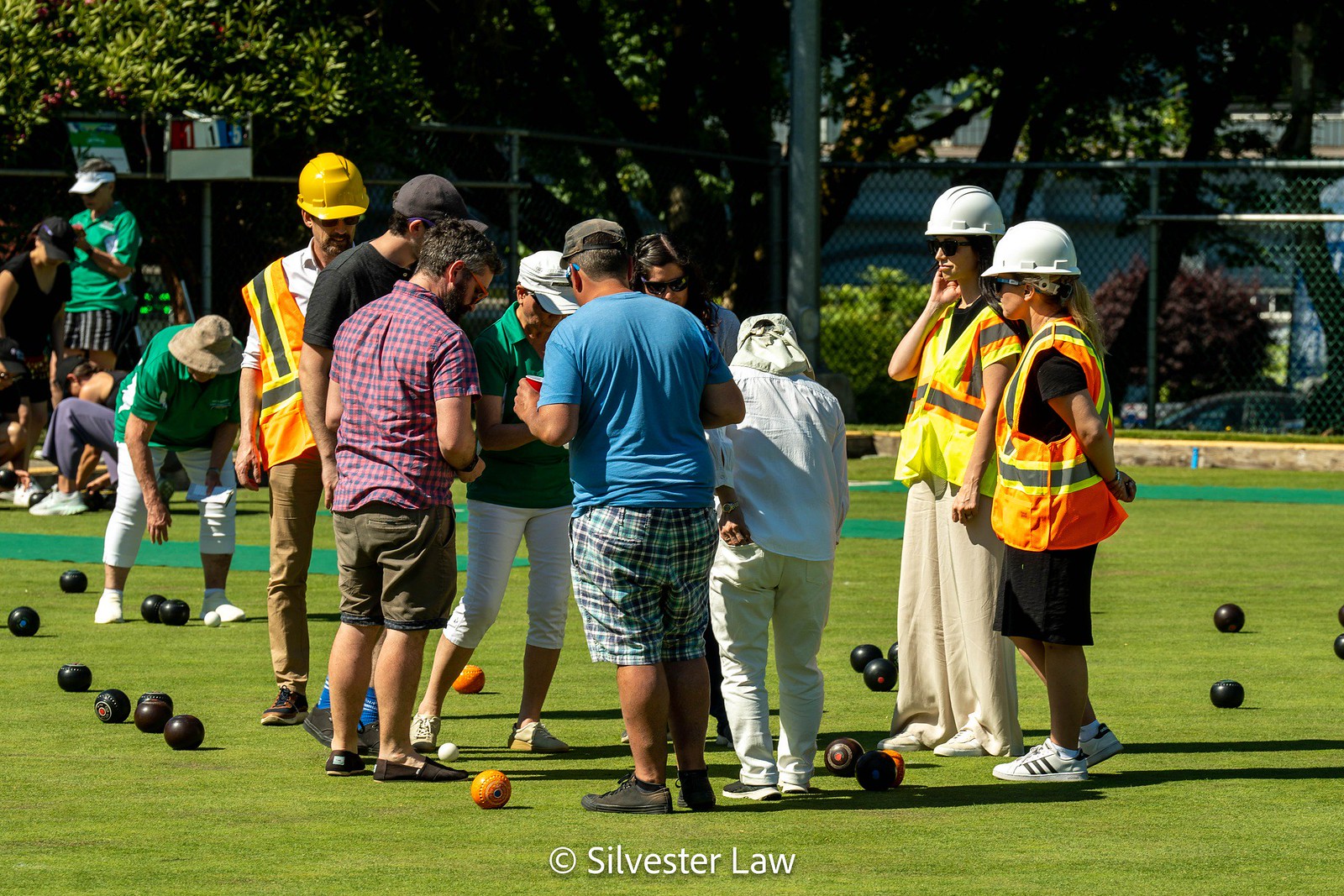In the image, a diverse group of people is gathered on a field bordered by leafy trees and a chain-link fence. The group includes individuals both in casual clothing and construction attire, with some wearing safety vests and white hard hats. At the center of the image, people are facing each other, seemingly focused on the ground, though it is unclear what exactly holds their attention. Scattered across the grass are several round balls, predominantly black, interspersed with orange ones. On the right side of the picture, a woman in a khaki hat, short-sleeved green shirt, and white capri pants is bending down to pick up one of the black balls. In the background, more people can be seen, some kneeling. Towards the bottom of the image is a partial label displaying a circle with a "C" and the text "Sylvester Law."